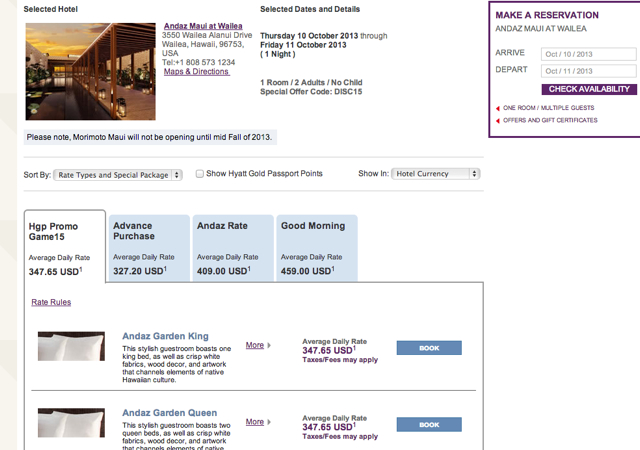The screenshot captures a webpage for a hotel reservation at the Andaz Maui at Wailea. The background is predominantly white with organized sections providing comprehensive information. 

At the top, there's a header labeled "Selected Hotel" accompanied by a colored photograph displaying what seems to be the hotel's exterior, possibly a patio area. Adjacent to the photograph, black text details the hotel's name "Andaz Maui at Wailea," its address, telephone number, and a link for maps and directions.

In the center section, there's information labeled "Selected Dates and Details." It specifies the reservation dates as Thursday, October 10th, 2013 through Friday, October 11th, 2013, for a one-night stay in one room for two adults, with no children. A special offer code "DISC15" is also mentioned.

On the right side, a black-outlined rectangle contains reservation specifics with black text on a white background. This section includes options to make a reservation with details such as "Andaz Maui at Wailea," arrival on October 10, 2013, and departure on October 11, 2013. It prompts the user to check availability for one room and multiple guests and offers information on gift certificates.

The bottom half of the screenshot continues with a white background, featuring sorting options for rate types and special packages. There's a segment for "Hyatt Gold Passport Points" and tabs labeled "HGP Promo," "Game 15," and "Average Daily Rate $347.65 USD," along with rate rules. Two photographs showcasing pillows on a bed indicate pricing for rooms with either a king or queen bed, both listed at the same rate. Additional tabs at the bottom include options for "Advanced Purchase," "Andaz Rate," and "Good Morning."